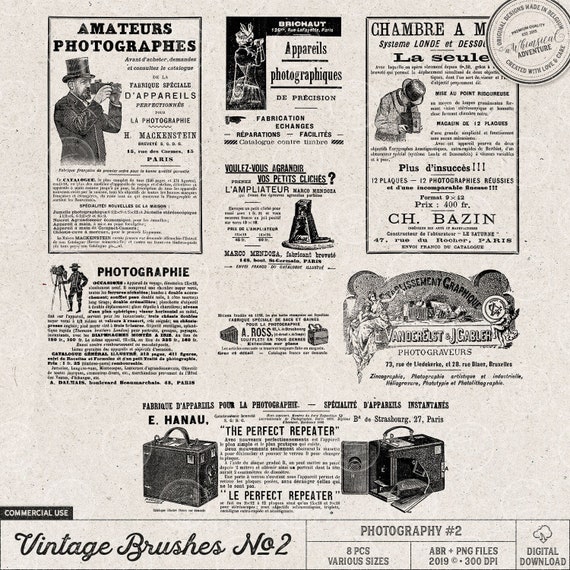Detailed Descriptive Caption:

The image is a black-and-white photograph that appears to be a page from an old catalog, possibly from the early days of photography. At the top, there is a bold heading that reads "Amateur Photographers." Below this heading, the image features a gentleman dressed in a black top hat and black jacket, holding an early camera model. Surrounding him is an assortment of textual descriptions.

Directly beneath, the prominent word "Photography" is displayed, accompanied by an illustration of a cowboy setting up an old-fashioned camera on a tripod. To the side of this image, there is a paragraph of text that is partially illegible.

In the central part of the page, the large, attention-grabbing word "Appareils Photographiques" is printed in French, translating to "Photographic Equipment." Adjacent to this text, there is a depiction of a black box with a person possibly holding a camera. 

Further to the right, another text segment begins with "Chambre A," followed by an unclear word, "Le Seul," and includes an illustration of a man wearing a hat and holding another vintage camera. 

At the bottom of the page, it states "C.H. Basin," perhaps indicating the name of a person or a business entity. Below this, the image details product information: "Commercial Use, Vintage Brushes, Number two, Photography, Number two, Eight pieces, various sizes, digital download."

In the middle of this lower section, the phrase "The Perfect Repeater" is highlighted, bordered by two black boxes on each side, which might represent camera equipment. The entire layout provides a captivating glimpse into vintage photographic tools and promotional materials, giving us nostalgia for the pioneering era of amateur photography.